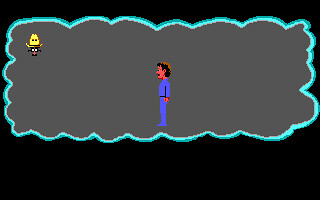The image depicts a retro-style, pixel art drawing, possibly a screen grab from an older video game or a modern piece emulating that aesthetic. The background is predominantly black, setting a stark contrast for the central turquoise cloud shape. Within this cloud, which features a gray inner background, stands a man viewed in profile, facing left. He has curly brown to black hair and a mustache, dressed in a matching blue long-sleeved shirt and pants. His arm is extended downward. In the top left corner of the cloud shape, there is an intriguing mix of quirky elements: an orange flame-like character with arms raised, two eyes, and a cowboy hat, which seems to have eyes of its own, beside a playful disguise featuring glasses, a fake nose, and a mustache. The overall effect is cartoonish and vividly detailed, capturing a sense of whimsical, nostalgic charm.